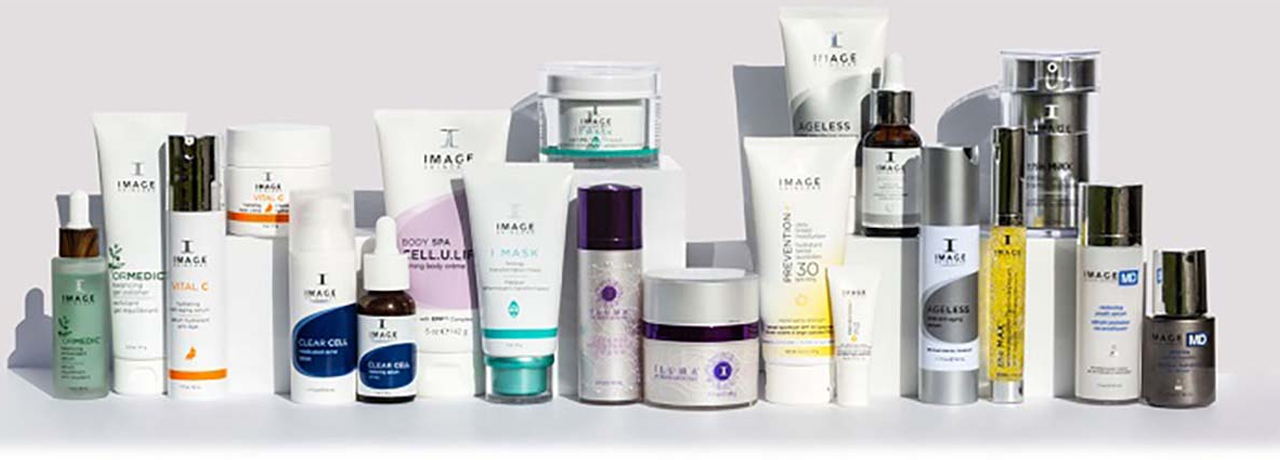The image depicts a meticulously arranged collection of skincare products set against a pristine white background, photographed from a front-facing viewpoint. The array of products includes a variety of bottles and tubes, predominantly white in color, accented with hues of gray, purple, and green. Displayed prominently on most of these containers is the brand name "Image," inscribed in black. The products feature labels with terms such as "ageless," "prevention," "clear cell," "cellulite," and "SPF 30," suggesting a broad range of skincare solutions including anti-aging, prevention, and treatment for various skin concerns. The overall composition and arrangement of the products hint at a professional photo shoot, designed to highlight the diversity and branding of the skincare line.